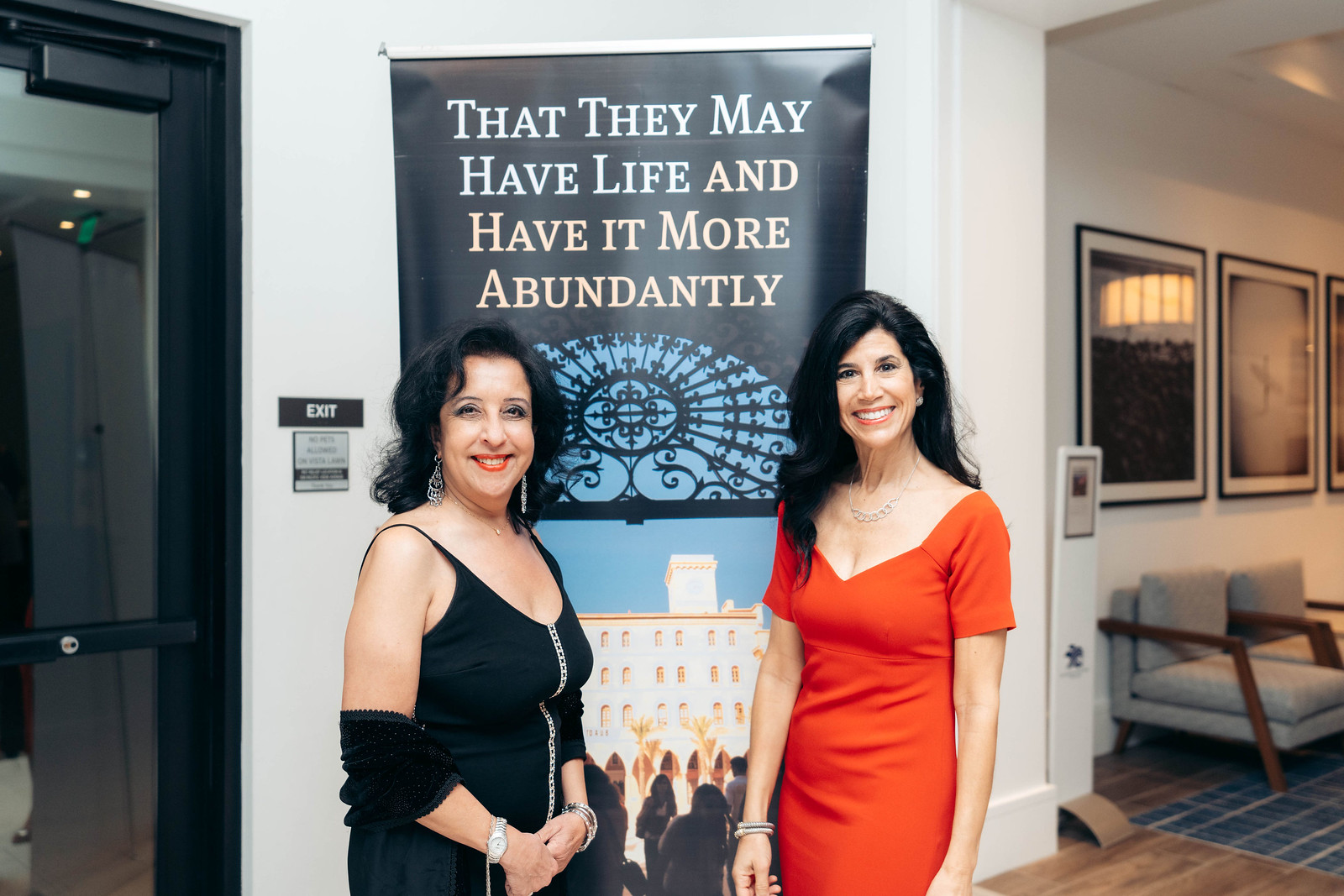This photograph captures two women posing cheerfully in front of a poster mounted on a wall inside a room. The woman on the left is attired in a black party dress with a shawl loosely draped around her mid-arms. She accessorizes with a silver watch on her right wrist and multiple bracelets on her left. Her black hair, slightly shorter than her companion's, frames her face, and she is wearing earrings. The woman on the right is dressed in a striking red party dress, featuring a low-cut neckline and short sleeves. She complements her outfit with a necklace, earrings, and two bracelets on her right wrist. Her black hair cascades past her shoulders.

Behind them, the poster features a notable quote in white text against a black background: "that they may have life and have it more abundantly." The poster also includes an image of a building under a blue sky, with additional figures visible. Positioned close to an exit sign near a glass door, the scene is part of a room designed as a lounge or waiting area. This space includes chairs, a blue carpet, and some paintings adorning the walls, contributing to a welcoming ambiance that frames the women's vibrant presence in the photograph.